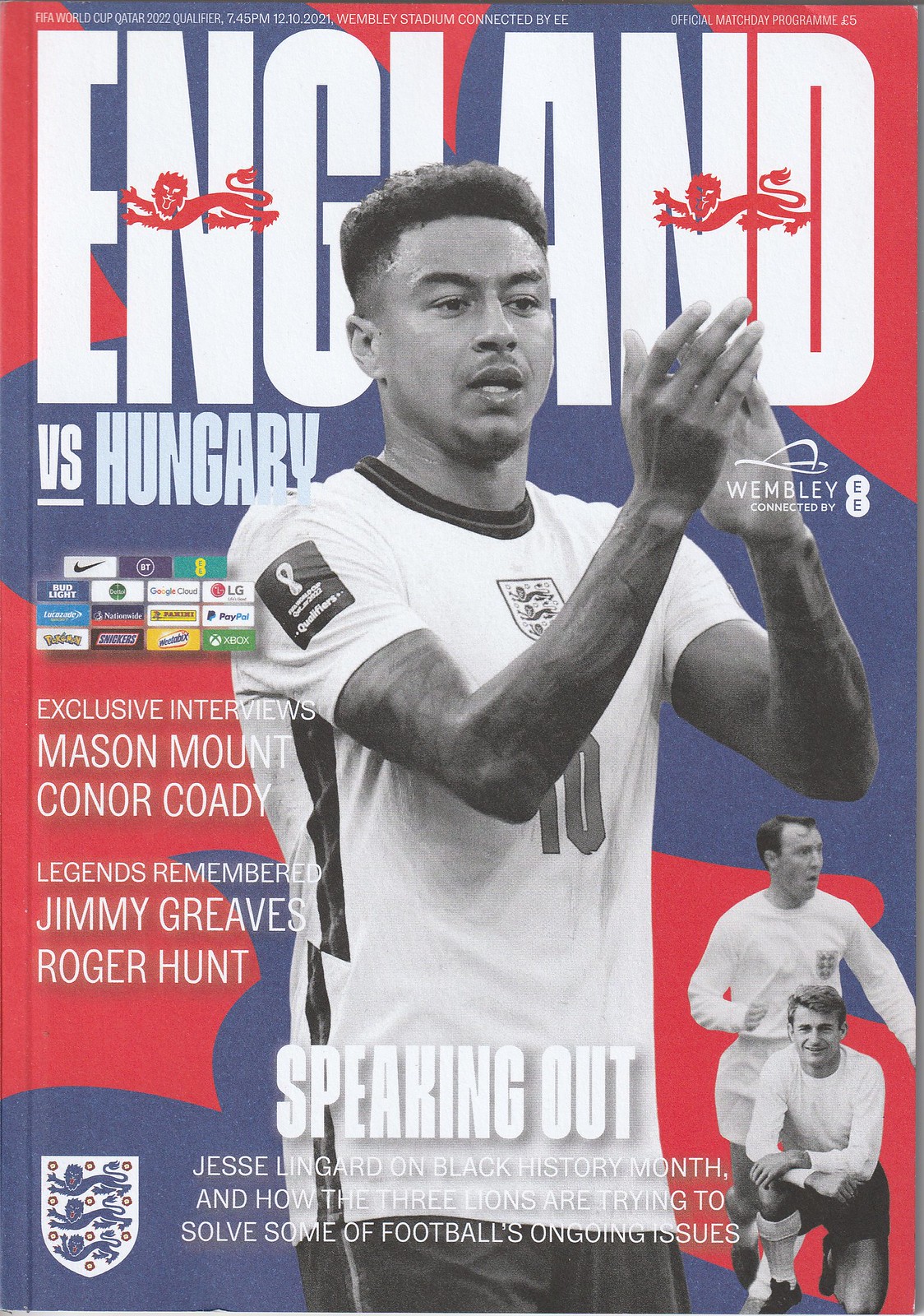The magazine cover prominently features a male soccer player clapping his hands, centered on the page, wearing a jersey with the number 10. The background is a striking mix of red and blue, with bold white text at the top reading "ENGLAND VS HUNGARY." To the right of the main player, there are two additional soccer players who seem to be from an earlier era. The cover includes several headlines: "Exclusive Interviews: Mason Mount, Connor Cody," and "Legends Remembered: Jimmy Greaves, Roger Hunt." At the bottom, there's a feature on Jesse Lingard discussing Black History Month and the efforts of the Three Lions to address ongoing issues in football. The cover also features various sports logos and branding, including the Nike logo and "Wembley connected by EE."